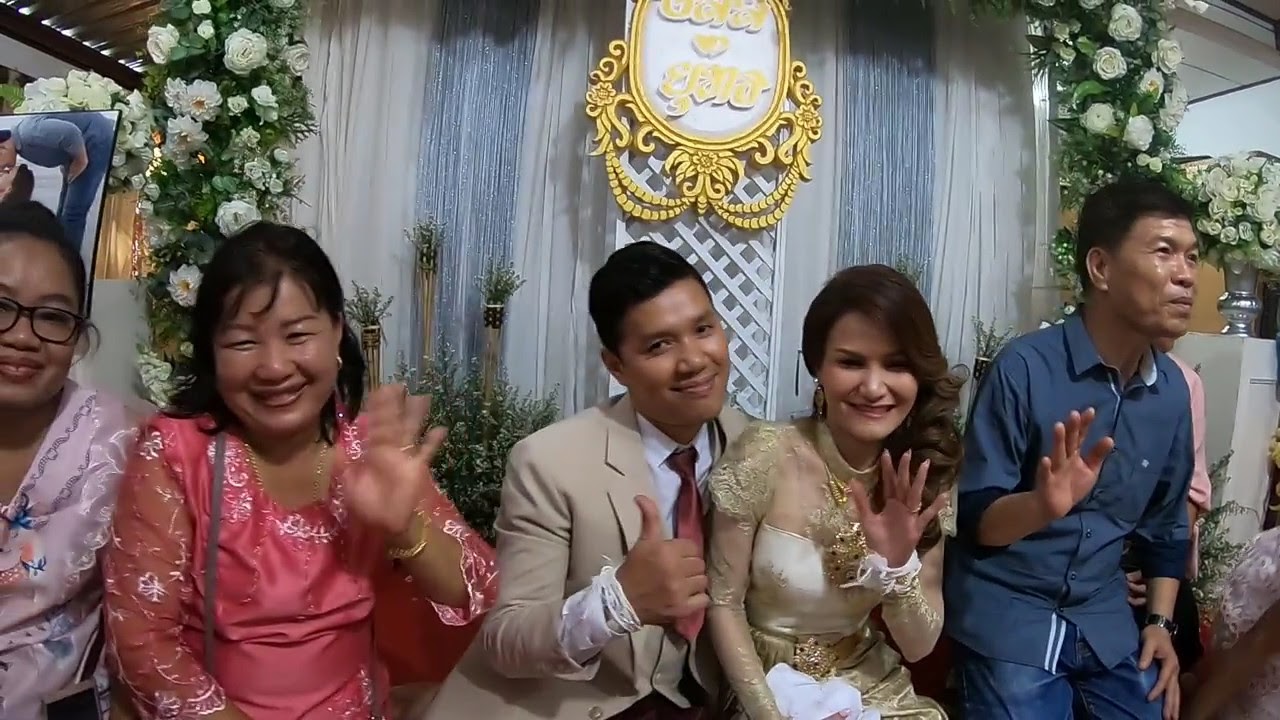In the center of the image are five people, all facing forward and smiling. The focal point is a man in a tan suit, white button-up shirt, and red tie, making a thumbs-up gesture with his right hand, where he wears a white string wristband. To his immediate left is a woman in a sheer, long-sleeved white and gold-decorated dress, holding a white cloth in her lap and also wearing a white string wristband. To her left is a man in a blue button-up shirt and blue jeans, appearing to be partially standing. Flanking the man in the tan suit on his right side are two older women. One of these women, wearing a pink dress with gold hoop earrings and possibly glancing at something off-camera, is seated next to another woman donning black glasses, a pink and purple dress, and waving enthusiastically. Behind them, an indoor setup featuring ornate decorations includes flowers, banners, and curtains in white and blue. A large, intricate, and partially obscured gold sign adorns the backdrop, heightening the celebratory atmosphere, which appears to be either a wedding or a party.